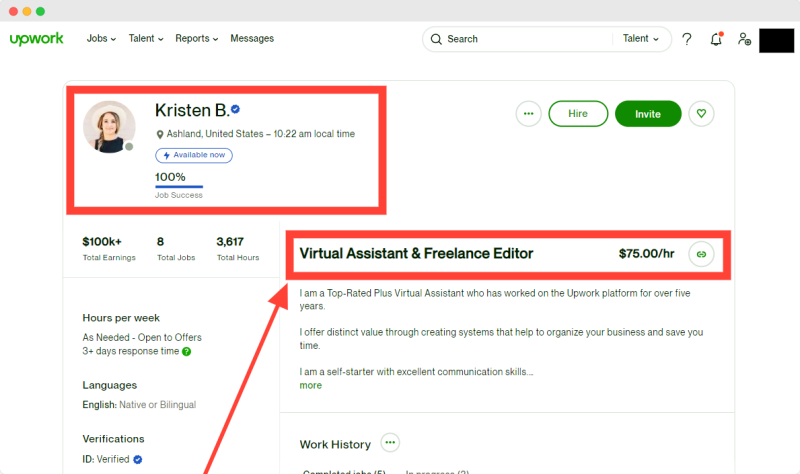Here is a detailed and cleaned-up caption for the image:

---

Screenshot of Kristen B.'s Upwork profile from Ashland, United States, taken at 10:22 a.m. local time. The top navigation tabs include Jobs, Talent, Reports, and Messages. Kristen boasts a 100% job success rate, with over $100k in total earnings across 8 jobs and 3,617 hours worked. She is currently available and open to offers as needed, with a response time of three or more days. Kristen is fluent in English at a native or bilingual level and has a verified ID badge indicated by a blue checkmark. She is a top-rated Plus virtual assistant and freelance editor, charging $75 per hour. Her profile description highlights her five-plus years on Upwork, emphasizing her expertise in creating organizational systems that enhance business efficiency. The description truncates with a "Read More" link for extended details. The profile also displays a partially visible work history section and features "Hire" and "Invite" buttons for prospective clients.

---

This caption captures the essential details while maintaining a clear and organized structure.